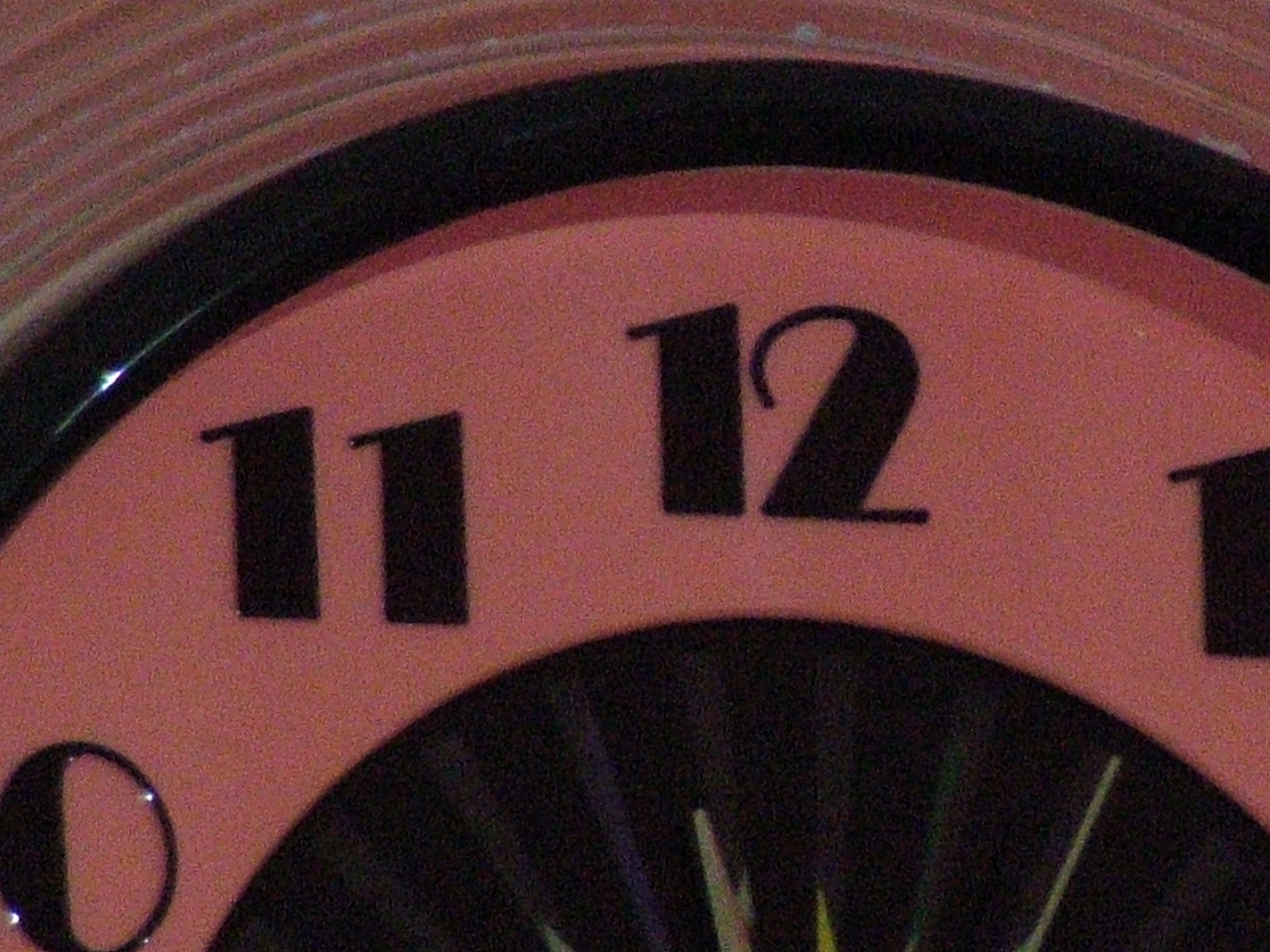This is a colour photograph showcasing a close-up of the top section of a clock face, rendered with a distinct filter. The clock's visible part reveals the numbers 11 and 12 prominently at the top, with the digits 0 and 1 intriguingly placed where the 10 and 1 should be, all set against a striking red backdrop. A shiny black rim outlines the clock, reflecting a small glint of light on the left side. Above this, a red curved textured surface adds intricate detail, resembling the ridged rim of a pottery plate. Beneath the numbers, partial clock hands, appearing yellow or green, point upward, contributing to a sense of movement, though it's difficult to distinguish hands from mere lines. The clock face exhibits a fan-like pattern with alternating dark and lighter segments of blue and grey, interspersed with some green elements. This intricately detailed area includes indents radiating towards the centre, enhancing the textured complexity of the timepiece.